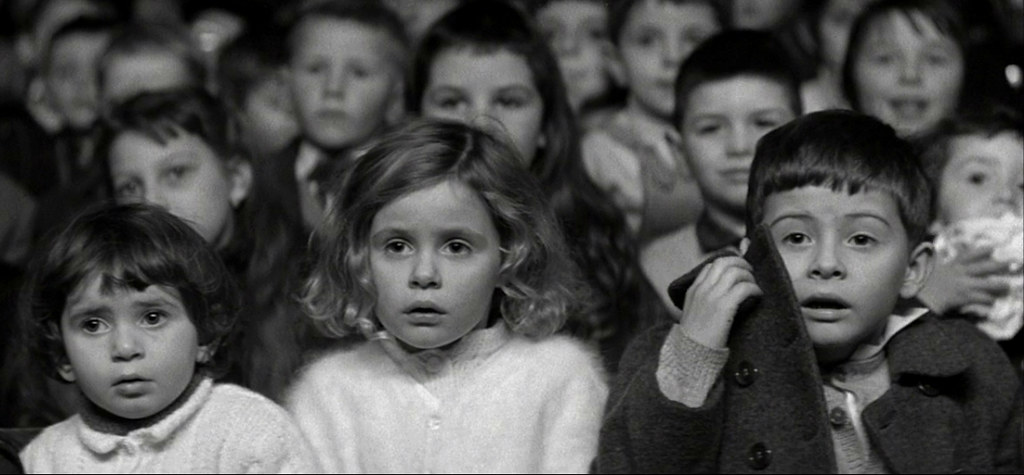In this black-and-white photograph, likely taken from the 1959 film "The 400 Blows," a group of children is shown intensely watching a puppet show, specifically a rendition of Little Red Riding Hood. The image is centered on three children in the front row, their expressions vividly capturing the moment. Situated on the left is a small girl with a short bowl cut, wearing a white sweater, looking apprehensive. Next to her is a slightly older girl with blonde wavy hair, also in a white fuzzy sweater, sharing a similar concerned expression. On the right is a boy with a short haircut, dressed in an old-fashioned long jacket with buttons. He holds the jacket up to partially cover his face, his mouth open in surprise. The background features multiple rows of other children, whose faces grow increasingly blurry with depth, reflecting the focus on the front trio. The photo encapsulates the children's absorbed and varied reactions, bringing a vintage, nostalgic essence to the scene.